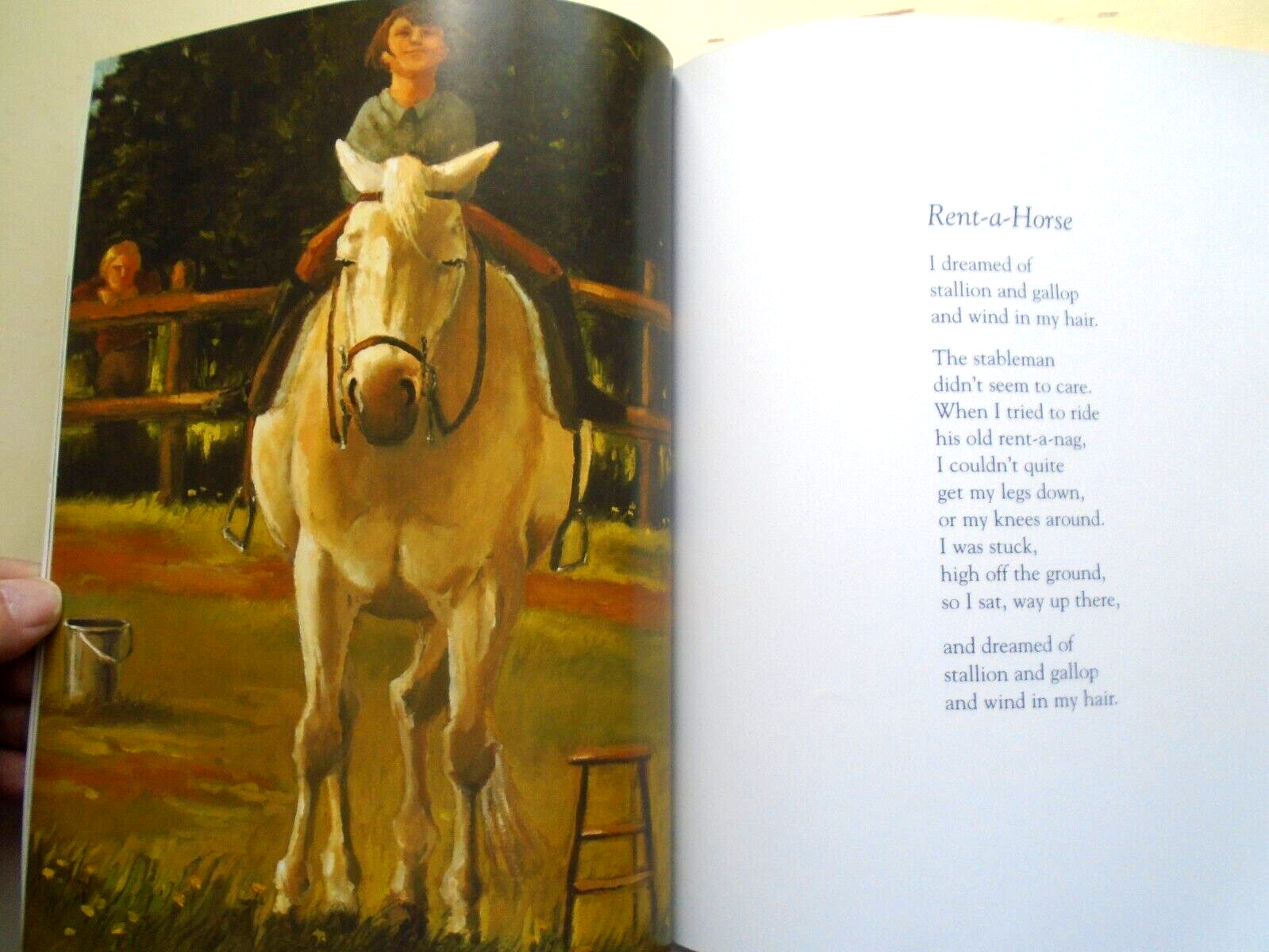An open book is held by a thumb on the left, revealing two detailed pages. The left page displays a vivid illustration of a child riding a friendly, white horse. The child, likely a boy, is attired in black riding boots, reddish-orange pants, and a blue collared shirt. The horse has closed eyes, a smiling demeanor, and a distinctive tuft of white fur on its forehead. In the scene, the duo appears to be in a corral with a wooden fence in the background, a stool nearby, and a pail on the ground. An older figure watches the child from outside the corral. The right page contains a poem titled "Rent-a-Horse," which includes three paragraphs of black text. The poem begins with the lines, "I dreamed of a stallion and galloped with the wind in my hair." The illustration’s colors predominantly feature greens and browns, enhancing the pastoral setting.